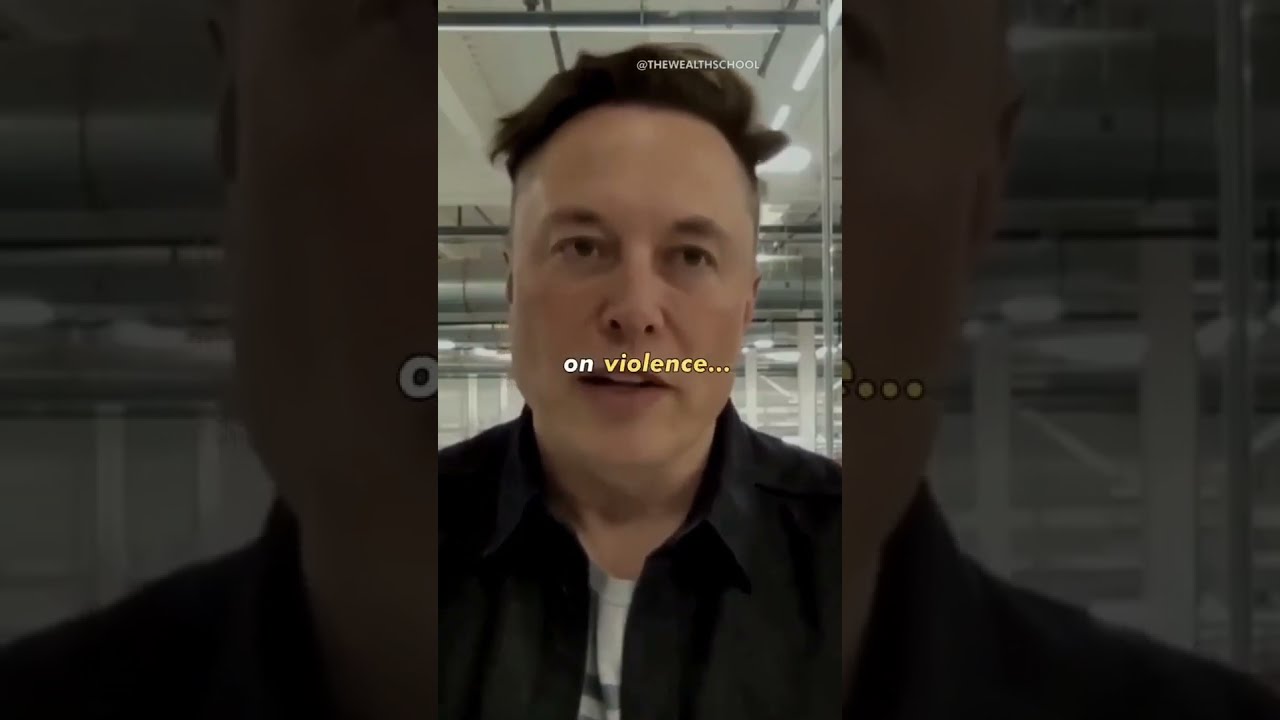The image is a large rectangular composite featuring Elon Musk, detailed with both photorealistic and partially blurred elements. The central portion of the image, forming a vertical strip from top to bottom, prominently showcases a clear photograph of Elon Musk. His brown hair is styled short on the sides and longer on top, revealing his forehead. He dons a black collared jacket over a white undershirt. His facial expression is neutral, yet slightly agape, showcasing his top front teeth.

Behind Elon, the background reveals an expansive warehouse setting defined by numerous white support beams and metal vents along the ceiling. Overlaying his face, the text "on violence" is written in lowercase; "on" appears in white, while "violence" is colored yellow. 

The left and right thirds of the image mirror the central segment but are zoomed in and darkened, making the colors less discernible. Additionally, small white text reading "At The Wealth School" is visible near the top right corner of the central photograph.